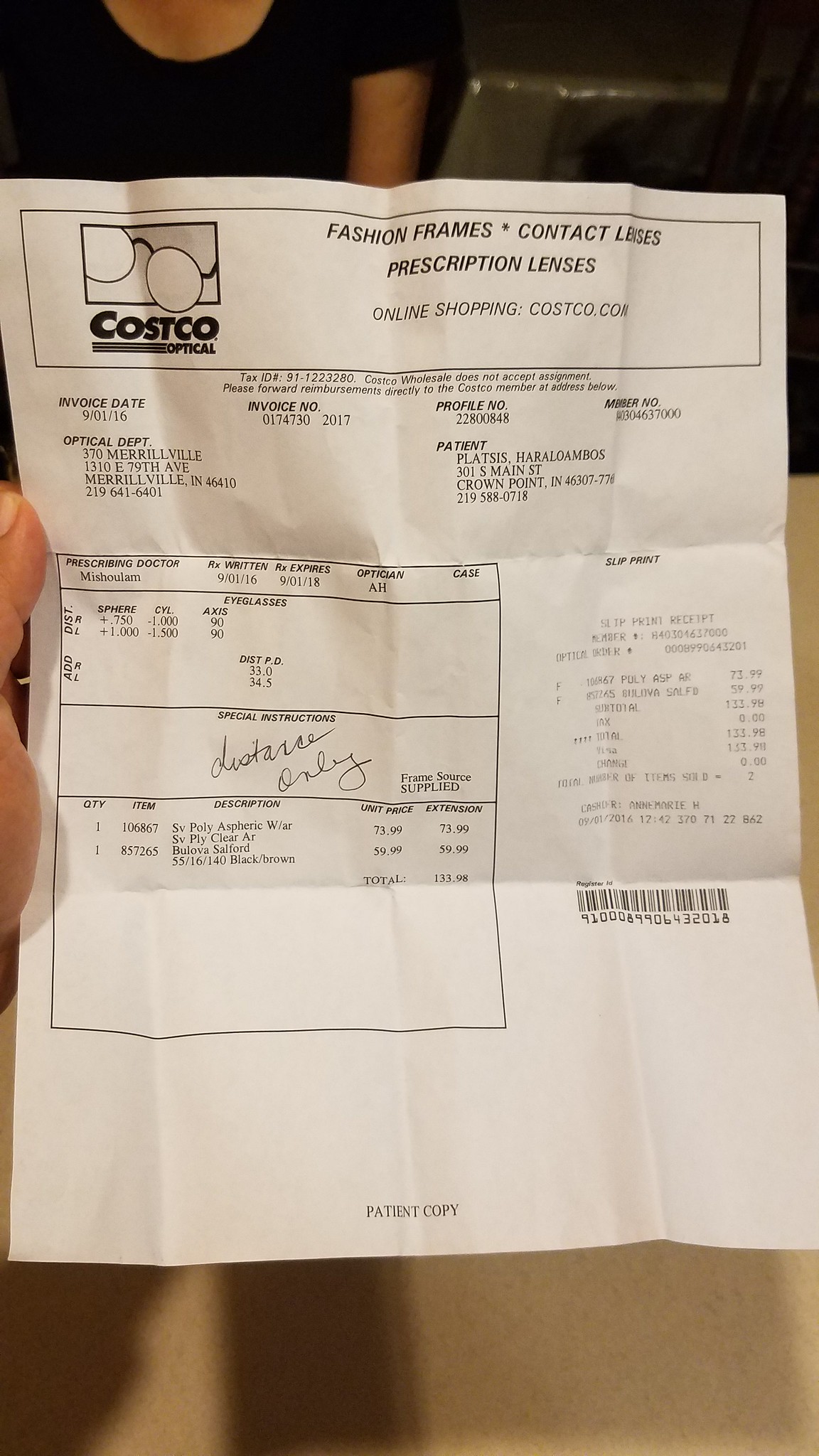Detailed Caption:
An invoice from Costco Optical, dated September 1, 2016, with invoice number 0174730-2017. The patient, Harlow Ablos Platisus, is listed with an address at 301 South Main Street, Crown Point, Indiana 46307, and a phone number of 219-588-0718. The invoice includes charges for fashion frames, contact lenses, and prescription lenses. It also references online shopping through Costco.com. The Optical Department is located at 370 Merrillville, 1310 East 79th Avenue, Merrillville, Indiana 6410, with a contact number of 219-641-6401. The invoice details the purchase of a couple of lenses and frames.